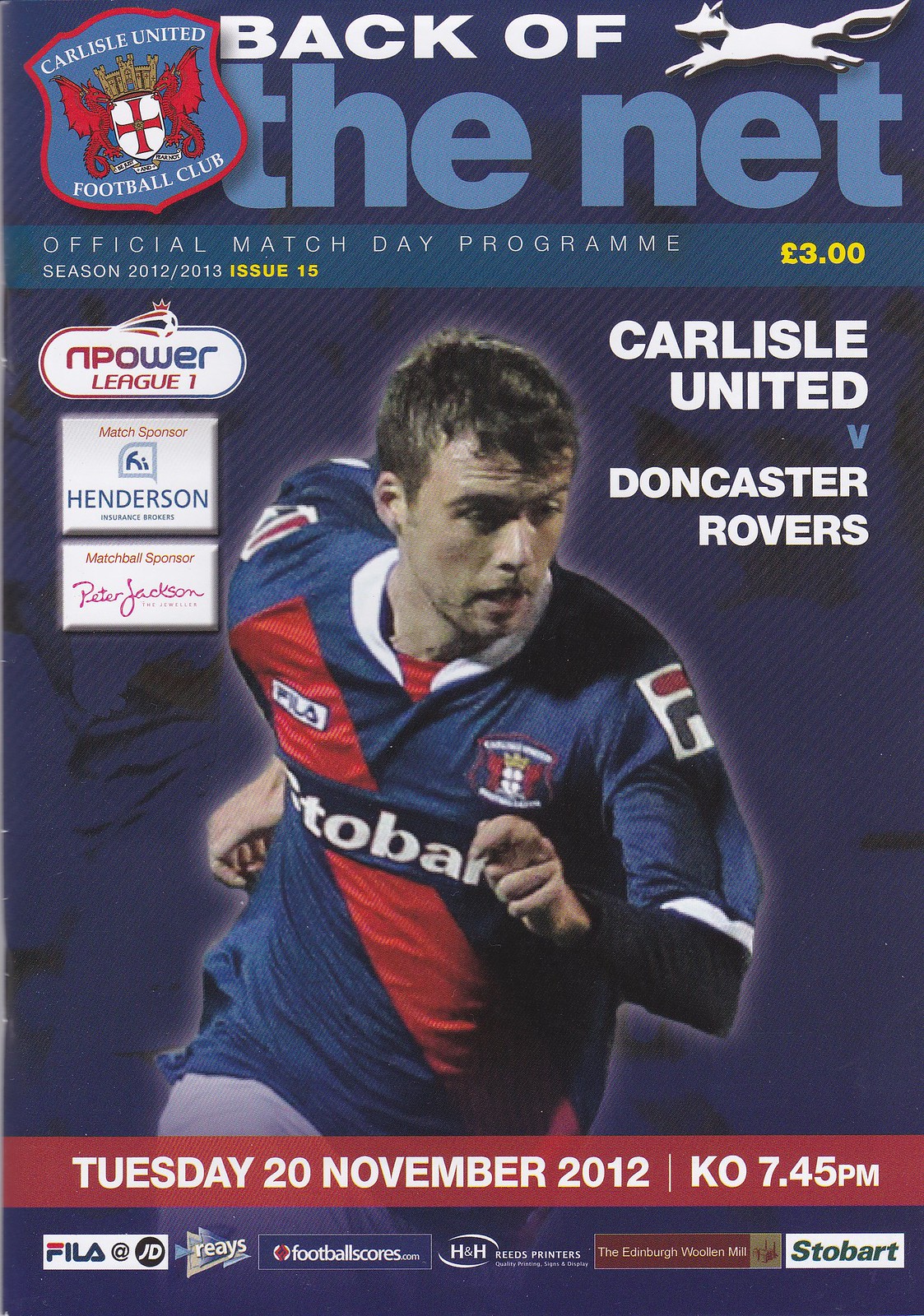The poster, predominantly a dark blue, serves as an official Match Day program for the 2012-2013 season, specifically Issue 15, priced at £3.00. At the top, in white letters, it proudly announces "Back to the Legends," and prominently displays the official insignia of the Carlisle United Football Club alongside a running fox. Central to the design is an eye-catching, large image of a player in mid-run, donned in a blue jersey with a striking red diagonal stripe running from his right shoulder to the lower left of the jersey. The player is surrounded by a white outline, giving him a glowing appearance as he wears a focused expression. On the right side of his head, it reads "Carlisle United v. Doncaster Rovers," while the left highlights "N-Power Elite One." Below, the date "Tuesday, 20 November 2012" and the kick-off time "KO: 7.45 pm" are displayed in red, clarifying the event details. Sponsors like Fila, Stobart, Henderson, and Peter Jackson are noted at the bottom, alongside other brands, contributing to the promotional essence of the poster.